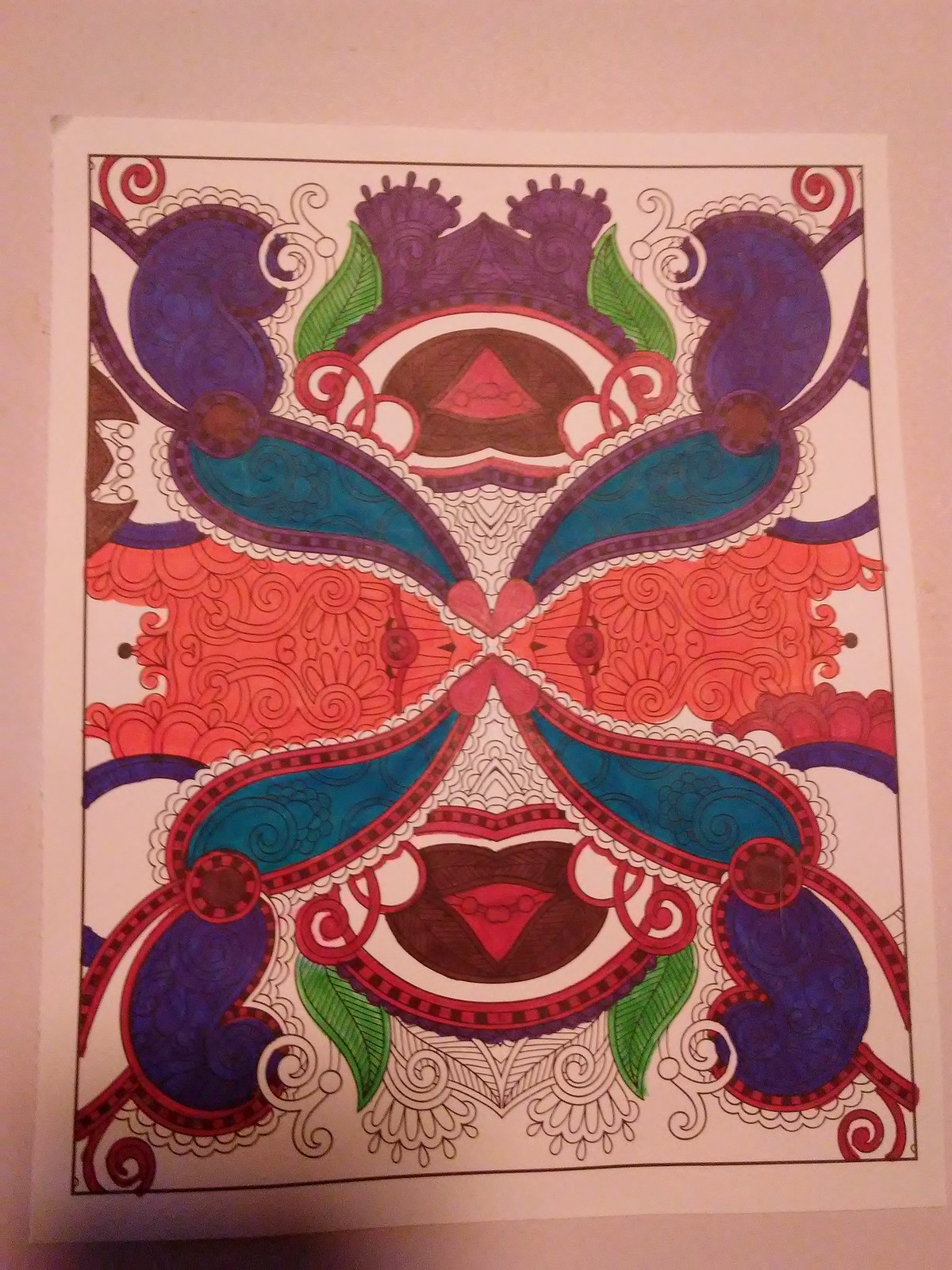This image showcases an intricate and symmetrically designed artwork, reminiscent of a mandala. It appears to be drawn on a white piece of paper and features a harmonious blend of shapes and patterns that mirror each other along both the horizontal and vertical axes. The central motif is composed of a combination of ovals and lines that fluidly extend outwards, gradually transforming into leaf-like shapes. The design radiates from a central point, transitioning through a captivating color gradient—starting with rich red hues at the core, shifting to vibrant turquoise, and culminating in deep purples at the extremities. The swirling patterns and meticulous detailing present a mesmerizing visual that embodies both complexity and balance.